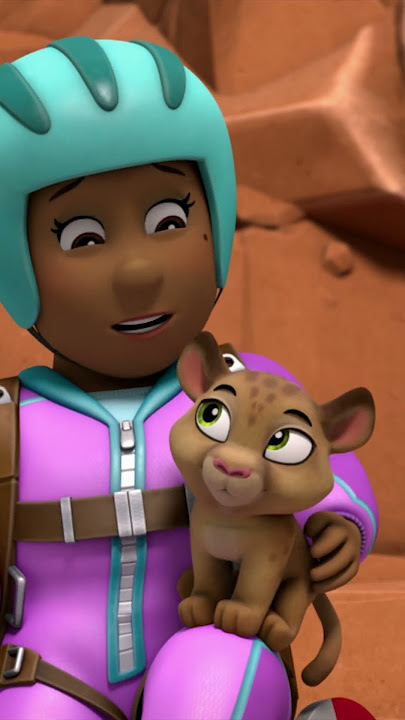This is a detailed screenshot from Season 13 of the children's animated show Paw Patrol. The image features an African American girl adorned in a teal helmet with darker green stripes and a purple jumpsuit with green and silver accents, which includes a brown harness across her chest and legs. The girl, seated on a rocky outcropping, is gently holding a small cub, possibly a baby leopard, on her knee. The cub, with distinct green eyes and brown fur marked with a few polka dots near its nose, looks up at her as she speaks to it. A terracotta-brown rocky formation forms the backdrop of this touching scene.